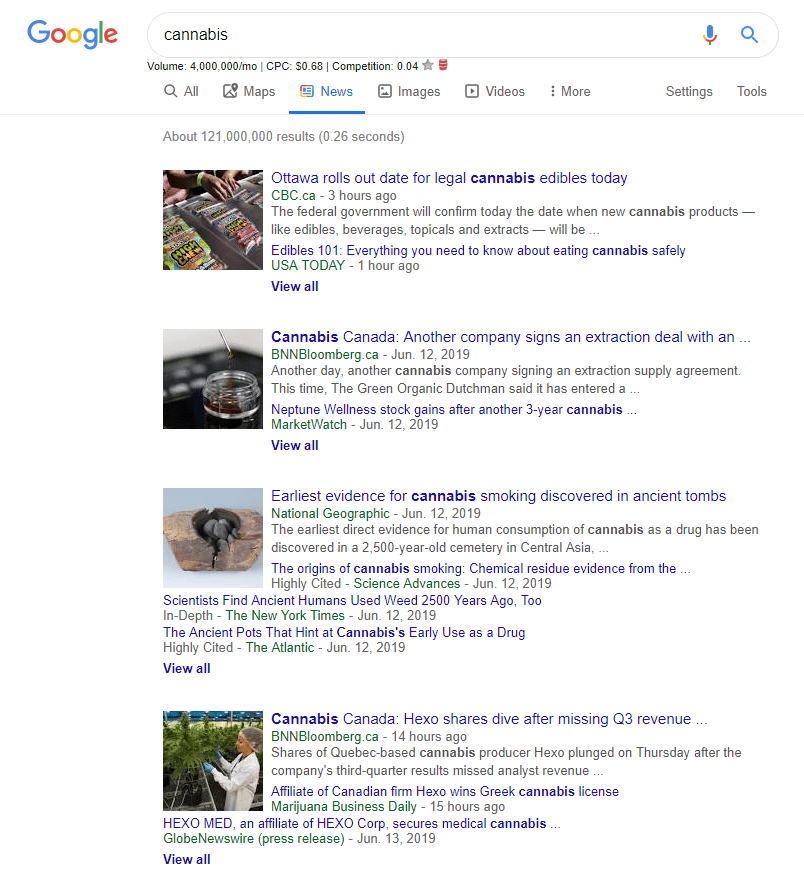A detailed Google search results page screenshot captures the scene. At the top-left corner, a distinctive Google logo is prominently displayed, featuring a large blue "G," a small red "o," a small yellow "o," a smaller blue "g," a small green "l," and a tiny red "e." Adjacent to the logo is the search bar, which has a white background and a subtle gray outline, rounded at both ends. Inside the search bar, the word "cannabis" is typed in black text. On the right side of the search bar, there is a microphone icon with a blue microphone and a multicolored stand, followed by a blue magnifying glass icon for the search function.

Beneath the search bar, small black text provides search metrics: "Volume: 4 million per month | CPC: $0.68 | Competition: 0.04," followed by a gray star icon and a red barrel icon. Below these metrics, various sections are listed in gray text accompanied by gray icons: from left to right, a magnifying glass icon for "All," an icon of a mountain with a geolocation pin for "Maps," a newspaper icon for "News" (this section is underlined in blue with the icon and text in color), an image icon for "Images," a video icon for "Videos," and three vertical gray dots for "More." On the far right are the options "Settings" and "Tools," without icons. 

A thin gray line underlines the "News" section, and to the center-left below it, light gray text states the total results: "About 121 million results (0.26 seconds)." Following this are the search results, where each entry has a blue title and an accompanying image on the left. Examples include:

1. "Ottawa rolls out date for legal cannabis edibles today."
2. "Cannabis Canada: Another company signs an extraction deal with N..."
3. "Released evidence for cannabis smoking discovered in ancient tombs."
4. "Cannabis Canada: Hexo shares dive after missing Q3 revenue..."

This screenshot provides a comprehensive and organized view of the Google search results for the term "cannabis", capturing both the interface and the content presented.